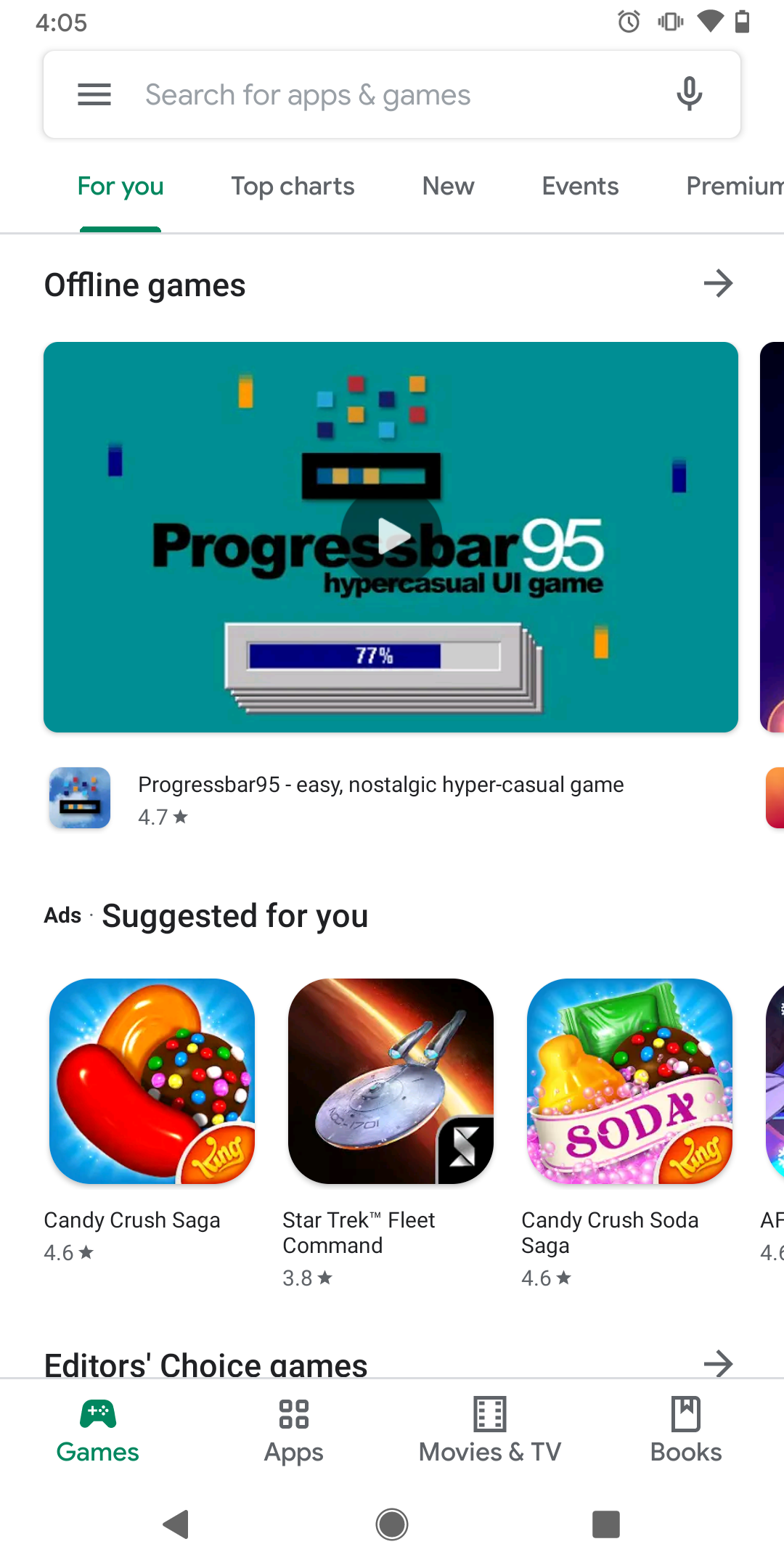This image features a white background. At the top, the time is displayed as 4:05. Below the time, there is a search bar with three horizontal lines on the left and a microphone icon on the right. Underneath the search bar, the words "For You" are written in green and underlined. This is followed by the options "Top," "Chart," "New," "Events," and "Premium" in a horizontal menu bar. 

There is a horizontal line dividing the sections, followed by a heading labeled "Offline Games" with a right arrow next to it. Beneath this, there is a bluish-green box, prominently displaying the title "Progress Bar 95." Within this box, there is a small gray progress bar showing 77% in blue. Next to this, on the left, there is a thumbnail image and text reading "Progress Bar 95 - Easy Nostalgic Hyper Casual Game" accompanied by a 4.7 star rating.

Further down, the section "Ads and Suggested for You" is presented, featuring various game recommendations such as "Candy Crush Saga" (4.6 stars), "Star Trek Fleet Command" (3.8 stars), and "Candy Crush Soda Saga" (4.6 stars). 

Below these recommendations, there is a section labeled "Editor's Choice Games," followed by categories titled "Green Games," "Purple Apps," "Purple Movies and TV," and "Purple Books." At the bottom, there is an icon with a left arrow, a circle, and a square, suggesting navigation options.